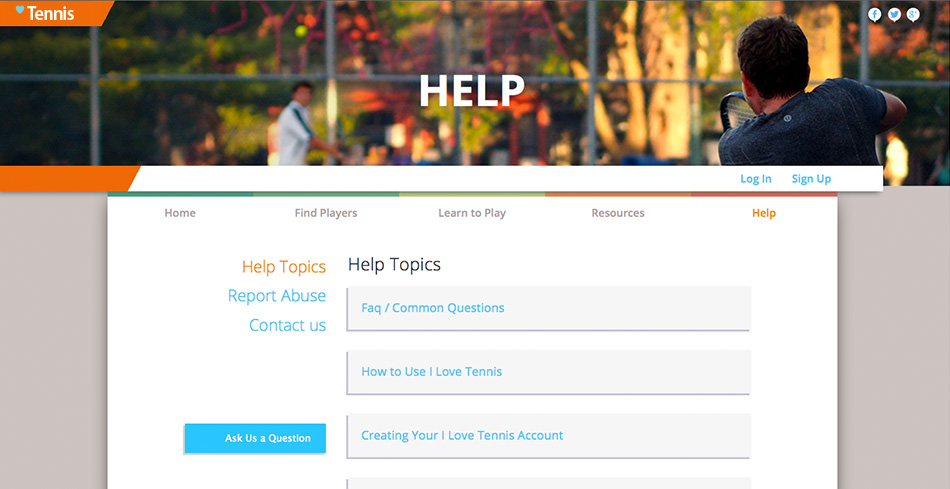This image is a detailed screenshot from a tennis-related website. In the upper left corner, there's a small orange tab labeled "tennis" in white text, with a tiny blue heart icon adjacent to it. A large banner spans the top third of the screen, featuring a dynamic photograph of two men engaged in a tennis match on a public court. One player, with his back to the camera, mid-swing with his racket visible, faces another player in a white shirt, blurred in the background. Both appear to be Caucasian with brown hair, and are playing on a court enclosed by a tall chain-link fence, with lush trees visible beyond. Below the banner, a navigational menu in a white box lists tabs for different sections: "Home," "Find Players," "Learn to Play," "Resources," and "Help." The "Help" tab stands out, highlighted in orange while the others are in gray. Further down, a section titled "Help Topics" provides blue clickable text links for various resources such as "FAQ," "How to Use I Love Tennis," and "Creating Your I Love Tennis Account," among others.